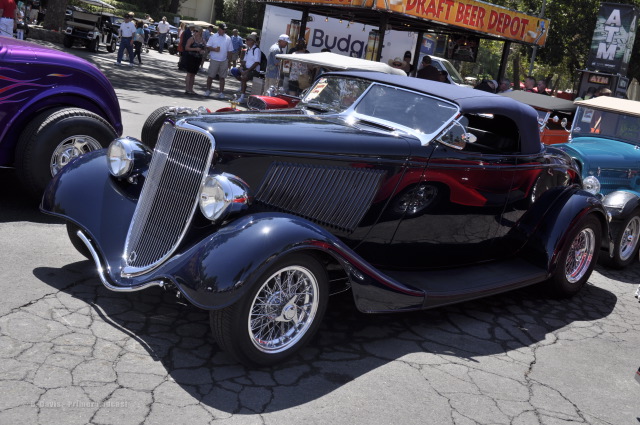The photograph captures a vibrant outdoor car show under a sunny sky, set against the backdrop of a quaint street with cracked pavement and patches of old brickwork. Dominating the image is a meticulously restored vintage roadster, painted in a strikingly dark hue that appears to be either black or a deep blue. This classic car, reminiscent of vehicles from a Dick Tracy comic or an early era Model T, features a long, tall grille with prominent metal spokes on its rims and side vents below the hood, suggesting it's likely a hot rod with a potential convertible soft top.

Surrounding the main attraction are glimpses of other classic cars, enhancing the nostalgic atmosphere. Directly behind the highlighted vehicle, you can spot a purple car with flames painted along its body, a red hot rod with a white soft top, a turquoise car with a white top, and an orange car with a black top. These cars are partially obscured but clearly add to the rich tapestry of the car show scene.

The car show is bustling with activity, as evidenced by the crowd of onlookers in casual summer attire—t-shirts and shorts—lining the sidewalk. They stand in front of a place called "Draft Beer Depot," prominently advertised by a yellow sign with red text. To the right, another sign indicates the presence of an ATM, and an adjacent establishment could be a movie theater, completing the lively, small-town setting. The combination of sunny weather, classic cars, and excited spectators creates a visually compelling and nostalgic scene.